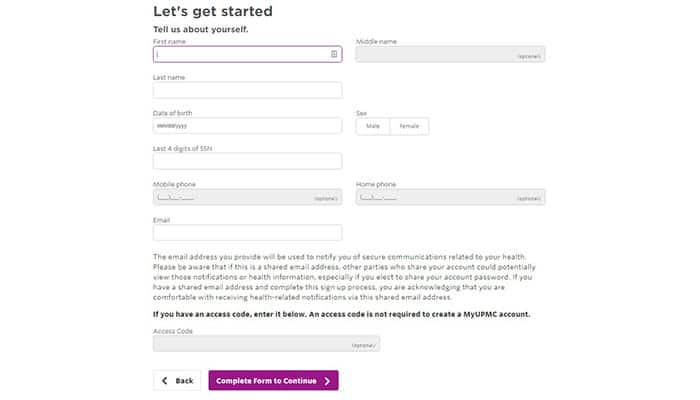The image depicts a web form titled "Let's Get Started" located at the top left in black font. Below this title, there's a prompt that reads, "Tell us about yourself." The form is organized into several sections with input fields for users to fill in their personal information.

1. **First Name**: A drop-down box with a white background.
2. **Middle Name**: A rectangular input box shaded in gray, positioned next to the first name drop-down.
3. **Last Name**: Located directly below the first name field, featuring a white input rectangle.

Beneath the last name field is another section for the user's **Date of Birth**, alongside a rectangular box for input. Adjacent to it is the **Sex** section with two small checkboxes labeled "Male" and "Female."

Below the date of birth section is a field for the last four digits of the user's **Social Security Number (SSN)**, followed by input boxes for **Mobile Phone** and **Home Phone**, both shaded in gray. Positioned beneath these phone number fields is a white input box for the user's **Email**. Adjacent to the email input is a disclaimer in smaller text, informing users that "the email address you provide will be used to notify you of communications related to your health."

Further down the form, there's a section in black letters that reads, "If you have an access code, enter it below. An access code is not required to create a myUPMC account." A shaded gray box is provided for the access code.

At the bottom of the form, there are two buttons:
- A small white rectangle with a black left arrow labeled "Back."
- A larger magenta maroon rectangle featuring a white right arrow labeled "Complete Form to Continue."

The overall layout is user-friendly, allowing for easy navigation and input of required information.